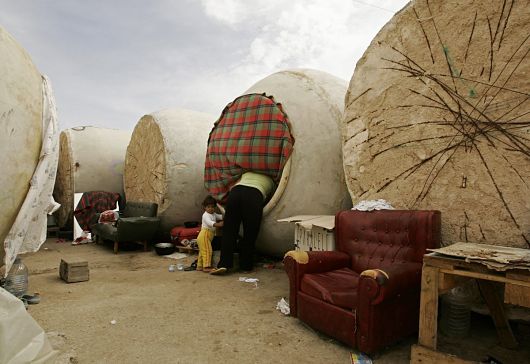The image depicts a makeshift camp that appears to be set in a developing country, possibly in the Middle East. The sky in the background is gray with fluffy clouds. Large cylindrical structures dominate the foreground, resembling gigantic ceramic urns or wooden pods, standing around ten feet tall. One cylinder has a large flannel blanket in red, green, and black draped over it, acting as a makeshift entrance. A person, dressed in a green shirt and black pants, is halfway inside this cylinder, while a young child with short dark hair, tan skin, barefoot, wearing a white shirt and yellow pants, stands nearby. Scattered around are remnants of daily life: a ragged red leather chair with bits of leather ripped off, revealing the tan insides; another green chair with wooden stool-like legs; a makeshift table constructed from pallets; an old barbecue; and boxes. The ground is sandy with garbage strewn about, further emphasizing the dire conditions of the setting.